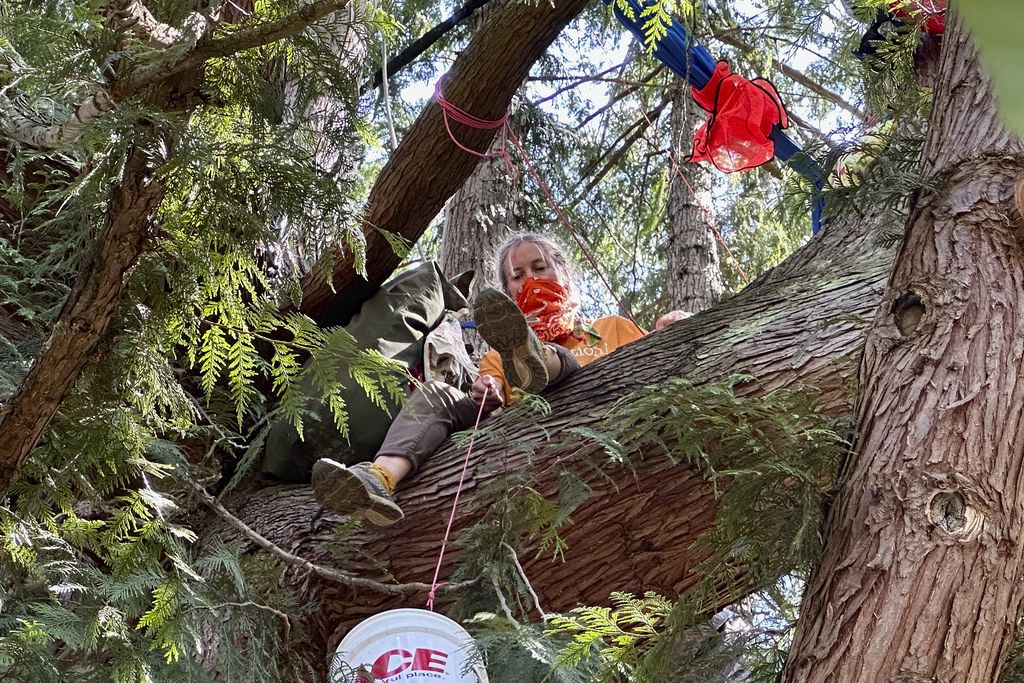In this image, a woman, who appears to be working or perhaps camping, is perched on a thick branch of a large coniferous tree. The perspective is from below, looking up at her. She has blonde, possibly tied, hair and is wearing an orange shirt with a red bandana covering her nose and mouth. She dons brown pants and tennis shoes, the bottoms of which are visible from this angle. A bucket with the letters "ICE" written in red dangles from a rope she is holding, and additional pink ropes are tied above her. Surrounding her are numerous branches adorned with various objects, including a red safety vest. The tree has rough bark and needle-like yet soft leaves, indicative of a pine. The sky is barely visible through the dense foliage.